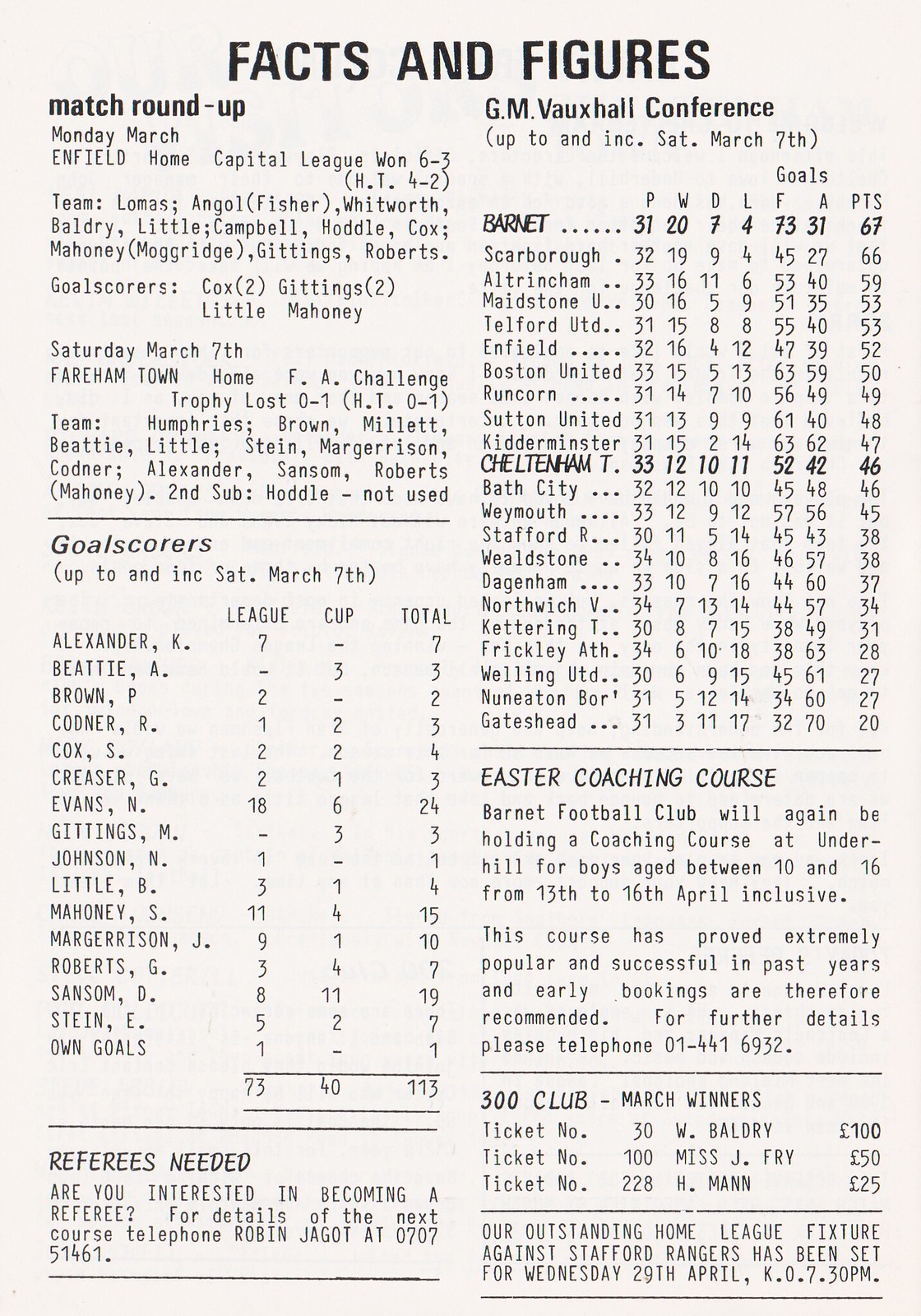The image portrays a section of a football club's newsletter or pamphlet, printed on an off-white background. At the top, the title "Facts and Figures" is prominently displayed, with detailed information organized in columns and rows about various soccer matches, players, and upcoming events.

On the left side, under the subtitle "Match Roundup," it provides details about a significant match held on Monday, March, at Capital One stadium, where the home team won 6-3. Listed players include Colton Lomas, Angelo Fisher, Whitford Valdary, Little Campbell, Hoodie Cox, Mahoney, Moodridge, Giddings, and Roberts, with goals scored by Cox, Giddings, Little, and Mahoney. 

Further below, it includes statistics up to and including Saturday, March 7th, for scorers across various matches. Names such as Alexander K., Beatty A., Brown P., and many others are listed with their respective league and cup goals, totaling a grand sum of 113 goals. Additionally, it notes a recent FA Challenge Trophy match against Farram Town, lost 0-1, with detailed line-ups including Humphreys, Brown, Beadle, Little, and others.

On the right side, the "GM Vauxhall Conference" section lists numerous teams like Barnett, with several columns for statistics labeled P, W, D, L, F, A, and PTS, each filled with respective figures.

Beneath these sections, there are notices for "Referees Needed," encouraging interested parties to contact Robin Jadl at 070-514-61 for the next course, and information on an "Easter Coaching" course for boys aged 10-16 to be held in Uphill from April 13 to April 16.

Towards the bottom, March winners of the "300 Club" are listed, with ticket numbers 3100 and 128, and names such as W. Baldry and Miss J. Fry, winning $100 and $50 respectively. Another section mentions an upcoming home league fixture against the Stadford Rangers on Wednesday, April 29th at 7:30 PM.

Overall, the pamphlet serves as a comprehensive summary of recent matches, player statistics, upcoming events, and additional club-related announcements.